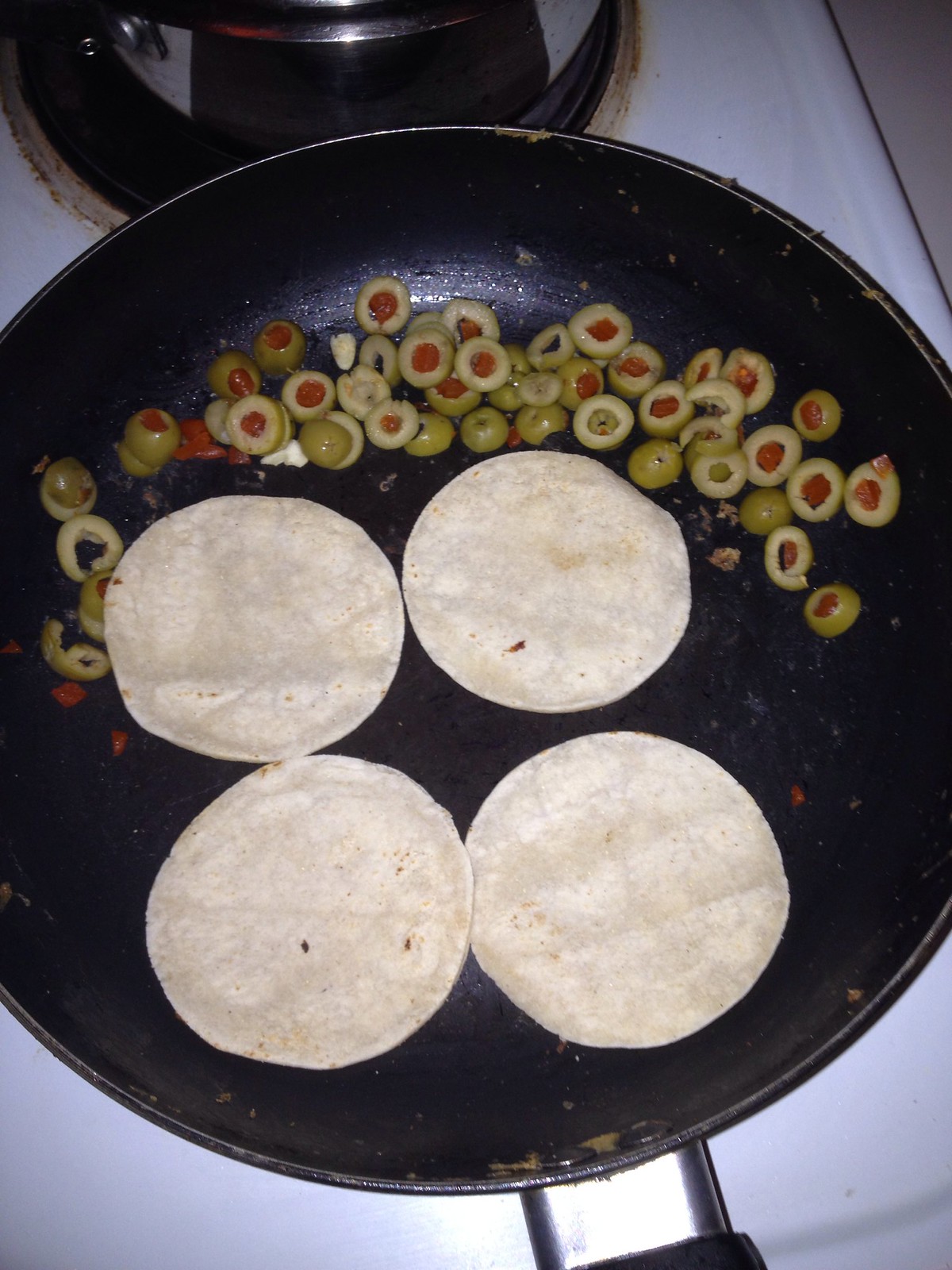This is a detailed color photograph looking straight down into a large, dark-surfaced skillet placed on a white porcelain electric stove with resistance coil burners. In the skillet, four flour tortillas, featuring light brown hues with scattered smudges and dark brown dots, are being warmed in a layer of shimmering cooking oil at the bottom of the pan. Along the upper edge of the skillet, sliced green olives stuffed with red pimentos lie, adding a splash of color. In the background, a pot or saucepan with a chrome-like appearance can be seen resting on another burner, and the stove top displays some smudge marks. The photograph also hints at the skillet’s handle peeking from the bottom right-hand corner of the image.